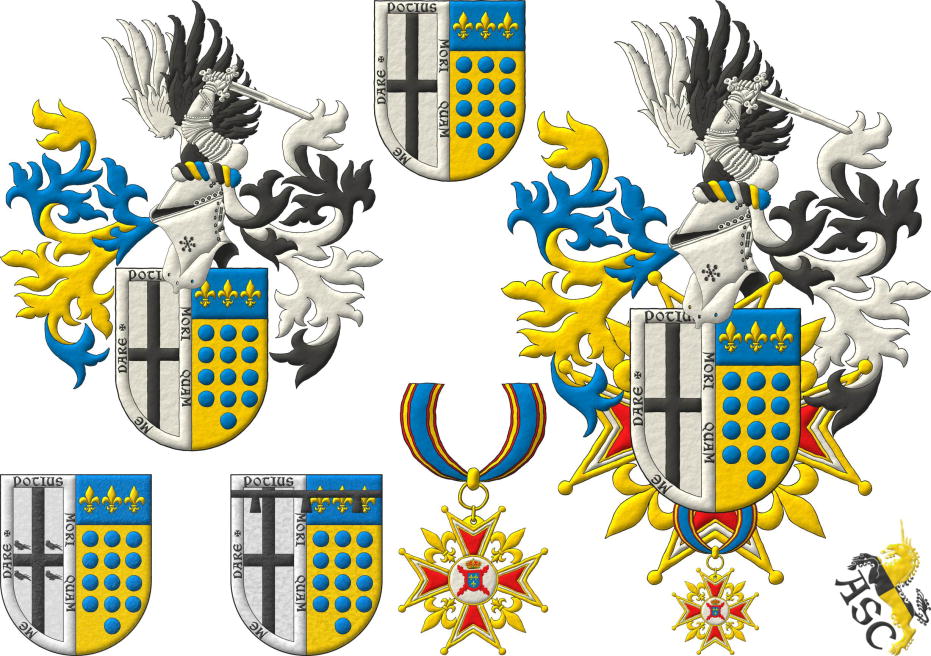The image showcases a meticulously detailed, square-shaped digital print that features an array of coat of arms and medals, all set against a plain white background with no borders. Central to the composition is a prominent shield divided into two distinct halves; the left half features a black cross on a gray background with the Latin phrase "Meus Dreik Politis Moriquam," while the right half is decorated with blue dots arranged in three vertical lines on a yellow background. This central shield design is flanked by larger versions that incorporate additional elements such as images of a knight, wielding a sword, and adorned with elaborate helmets from which gray, white, blue, and yellow feathers protrude. 

Identical shields appear in both the upper left and right corners, while smaller variations of these shields with slight design differences, particularly in the positioning of the black cross and the number of blue dots, are located in the lower left corner. In the lower middle section, a star-shaped pendant hangs, adding to the regal theme. Dominating the lower right corner is a golden unicorn clad in black armor on its back, tail, and front legs, with the inscription "ASC" beneath it. This visually rich collection evokes the grandeur of royal family crests and medieval heraldry, combining symbolic icons with exquisite detailing.